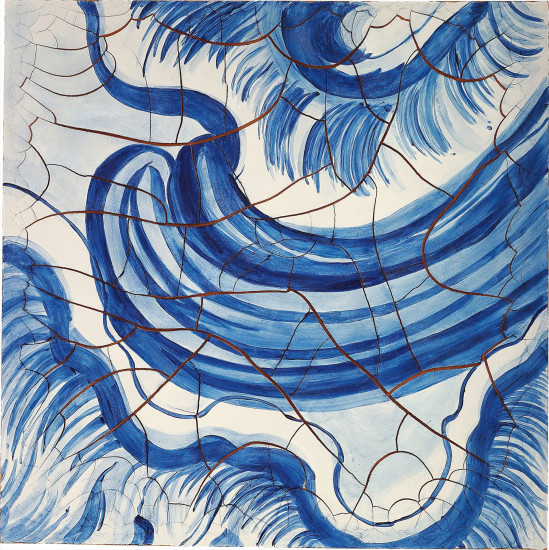This image resembles an abstract painting with a predominant white background overlaid with intricate blue and brown elements. The blue accents, reminiscent of royal blue paintbrush strokes, form various patterns including swirls, wavy lines, and hair-like textures, evoking a sense of movement across the vertical rectangular canvas. The blue elements are intricately layered, creating a fur or eyelash appearance. Interspersed among these blue details are crack-like brownish-red lines that lend a rust-colored accent to the artwork, giving it a vintage, porcelain-like quality similar to Dutch ceramic designs. The overall impression is of a meticulously detailed, abstract composition that harmoniously blends these colors and textures.